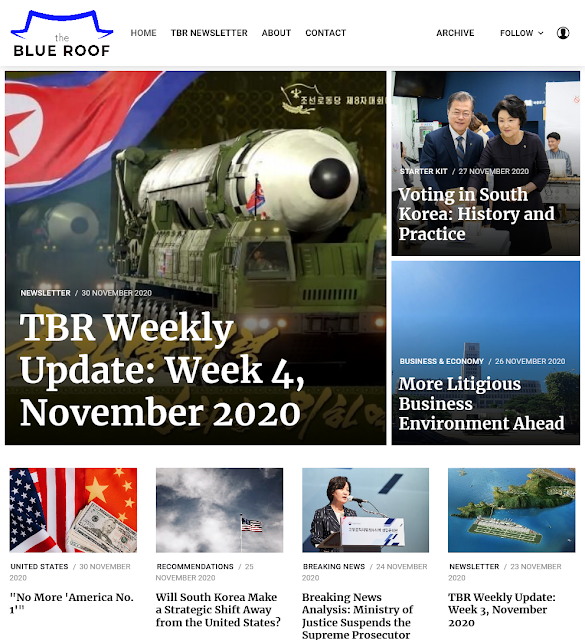This screenshot captures a detailed view of a news website named "The Blue Roof," prominently displayed in the upper left-hand corner. The top navigation menu hosts several options: Home, The Newsletter, About, Contact, Archive, and Follow. Beneath the menu, there are multiple images accompanied by clickable links directing readers to various news stories. 

The central and most prominent feature is a large image headlining the story titled "TBR Weekly Update Week 4, November 2020." To its right, a secondary clickable story is labeled "Voting in South Korea: History and Practice." Below these primary stories, there is an additional piece titled "More Litigious Business Environment Ahead."

Further down the page, four smaller images line the bottom, each linked to different news articles. The first article is labeled "No More America Number One," followed by "Will South Korea Make a Strategic Shift Away from the United States?" The final two stories are not specified. Based on the contents and focus of the articles, this appears to be a Korean news site.